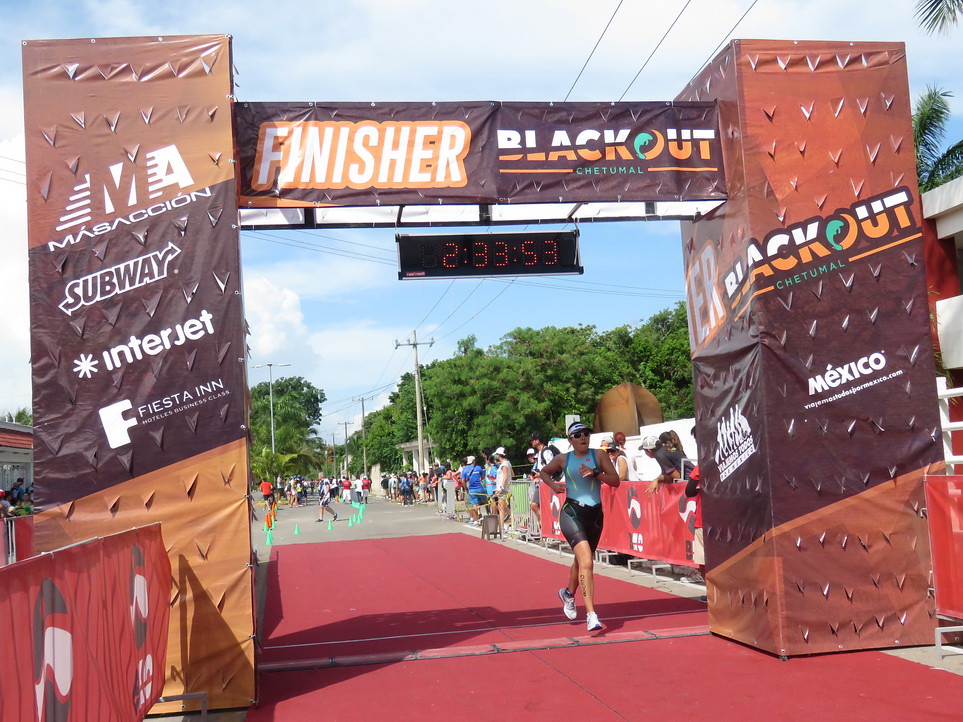The image depicts the thrilling moment of a marathon race finish line, where a solitary runner, who appears to be a woman, is crossing the line with a recorded time of 2 hours, 33 minutes, and 53 seconds displayed prominently above her on a digital clock. The finish line is vibrant with a red carpet surface stretching ahead, accompanied by spectators cheering on both sides of the route. The runner, identifiable in a blue top, black pants, white shoes, and possessing tanned legs marked with a race number, is set against a backdrop featuring a clear blue sky and lush trees. The scaffolding around the finish line is wrapped in tarpaulin, emblazoned with various sponsor logos including Massacion, Subway, Interjet, Fiesta Inn, and the country of Mexico. The top of the scaffolding proudly displays the words "Finisher" and "Blackout Chetumal". Additional small wording on the tarpaulin is present though not clearly readable in the image.